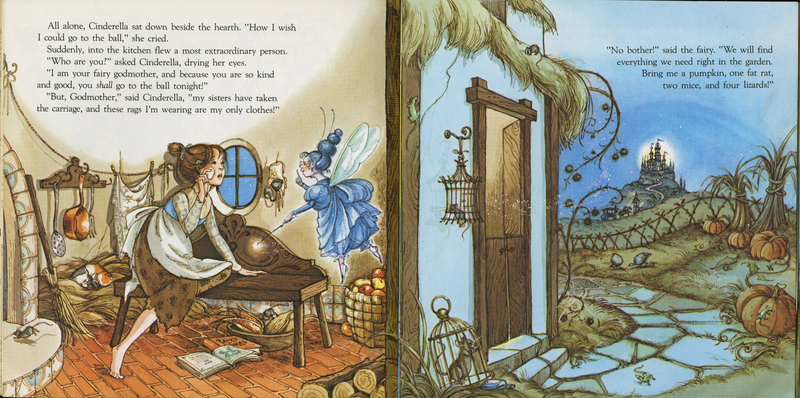This illustration from an open book features two panels depicting scenes from the fairy tale Cinderella. In the left panel, Cinderella, a young girl with brown hair tied in a bun, sits on a wooden bench near the hearth, wearing a brown dress with a white apron and a bluish-white top, and is barefoot. She gazes toward the right where a blue fairy with transparent wings and moth-like antennae hovers. The fairy, holding a wand in her left hand, speaks to Cinderella with a finger raised. The background includes laundry hanging on a line from the left wall to a window near Cinderella's face, a mouse headed toward the hearth, cooking pans on the wall, apples in a basket, and lumber in the right corner. Above Cinderella, the text reads: "All alone, Cinderella sat down beside the hearth. 'How I wish I could go to the ball,' she cried. Suddenly into the kitchen flew a most extraordinary person. 'Who are you?' asked Cinderella, drying her eyes. 'I am your fairy godmother, and because you are so kind and good, you shall go to the ball tonight.' 'But godmother,' said Cinderella, 'my sisters have taken the carriage, and these rags I'm wearing are my only clothes.'"

In the right panel, the scene shifts outdoors under a moonlit sky. The blue fairy instructs Cinderella, "No bother," said the fairy, "We will find everything we need right in the garden. Bring me a pumpkin, one fat rat, two mice, and four lizards." The setting features a quaint house with a blue stucco exterior and a straw roof. Nearby, pumpkins grow in the garden alongside corn stalks. By the door, a rat sits in a cage on the ground, while a mouse hangs in another cage near the entrance. The door itself has split panels with flagstone steps leading up to it. Vines climb up from the ground, and in the distance, a winding road leads to a castle perched on a hill, illuminated by the light of the moon. A small carriage can be seen traveling toward the castle.